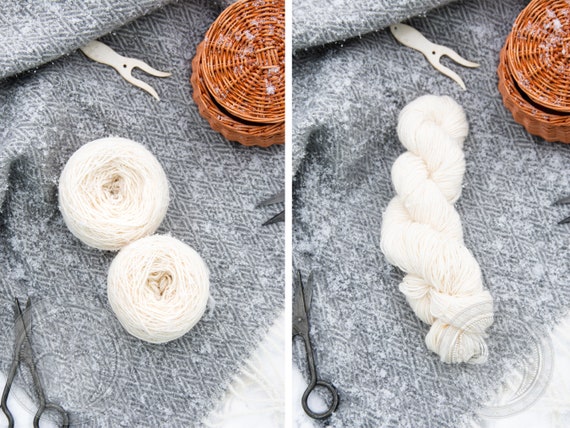The image features a detailed and cozy craft scene split vertically into two sections. Both parts share a textured gray background, possibly a knitted blanket or afghan, serving as the base for the displayed items. On the left side, two balls of off-white yarn sit prominently, accompanied by a pair of rusty black metal scissors positioned on the bottom left. Above the yarn, a white hook tool lies, potentially used for manipulating the yarn or cloth. The right section showcases similar elements including the black scissors and white tool, but with a transformation: the yarn has been intricately braided into a thick plait, resembling a pretzel rope. A small brown wicker basket with an open, upside-down lid rests towards the top right of both images, adding a rustic touch to the scene. The overall composition suggests a “before and after” snapshot of an artistic yarn project.